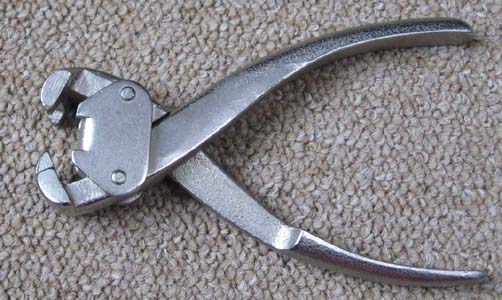This is a close-up, rectangular landscape photograph of bullnose pliers lying horizontally on a light brown, matted-down carpet. The handle of the pliers extends to the right side of the image, while the clamping end is positioned towards the left. The stainless steel pliers feature a thick, heavy front with two curved, flat ends that slightly part from one another, echoing the likeness of a bug's mandibles. Two visible rivets hold the handles together, and the entire metallic silver tool spans almost the entire frame, with the top handle very close to the top right corner and the bottom handle near the bottom right corner of the image.